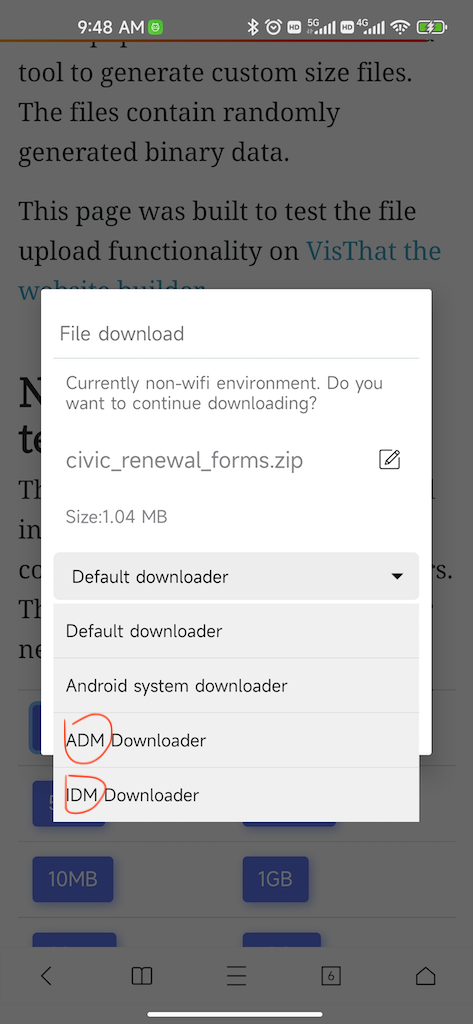In this screenshot, captured from a phone, the top area is grayed out, but still legible. The time displayed is 9:48 AM. Several icons are visible, indicating that Bluetooth, alarms, Wi-Fi, 5G, 4G, and the battery are all active.

A pop-up notification reads: "File Download. Currently in a non-Wi-Fi environment. Do you want to continue downloading?" Below this message, there's a zip file mentioned with a size of 104 MB, and three download options: Default Downloader, ADM Downloader, and IDM Downloader. Both ADM Downloader and IDM Downloader are circled in red.

In the background, there are blue squares with text: one indicating "10 megabytes" and another "1 gigabyte." Additionally, three more blue squares are partially visible beneath them. Next to these blue squares, a paragraph starts with the text: "Tool to Generate Custom Size Files. The files continue randomly generated in binary data. This page was built to test the File Upload functionality on this laptop."

The screenshot captures a detailed interaction with file download prompts and background information on a file generation tool.